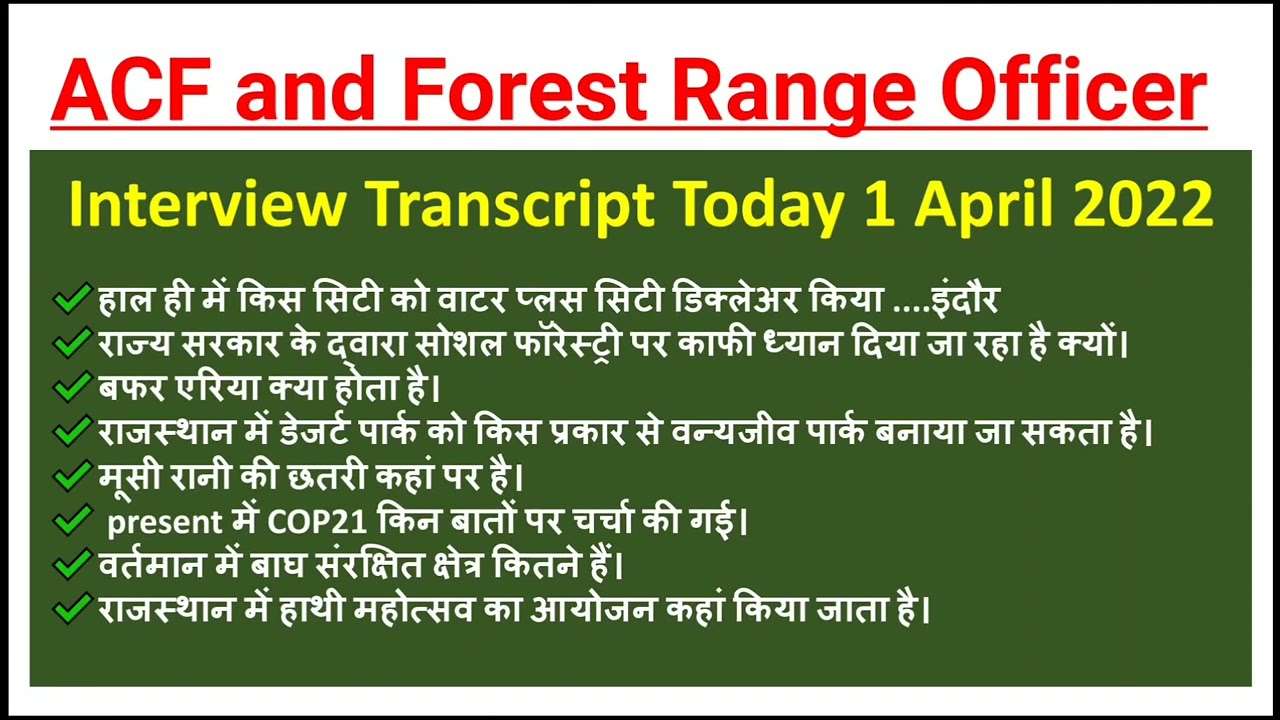The image appears to be a PowerPoint slide with a thin black border encasing a white background. At the top of the slide, bold red letters, underlined, read "ACF Enforced Range Officer." Below this heading, a dark green rectangle features yellow text that says "Interview Transcript Today, 1 April 2022." Within this green rectangle, there are multiple green check marks, each followed by white text written in what seems to be an Indian script, possibly Hindi. Among the foreign characters, occasional English words such as "present," "cop," and "21" are discernible. The check marks and the contrasting text format stand out clearly against the dark green background, making the details prominent.